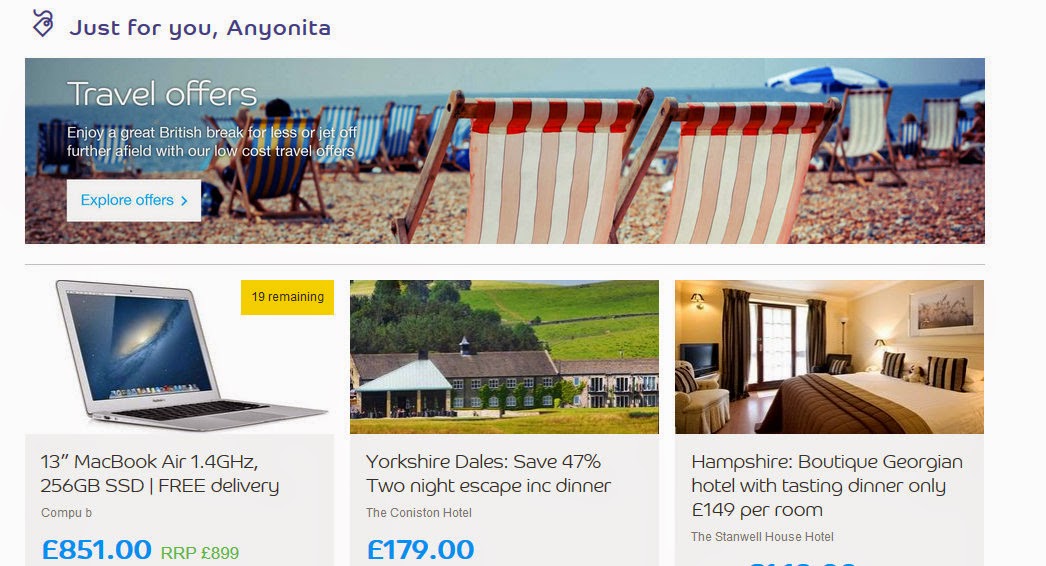The webpage features a prominently displayed long rectangular image at the top, followed by three smaller images arranged in a row beneath it. In the upper left corner of the page, the text "Just for you Anonita" is written in dark blue. 

The large top image showcases a picturesque beach scene, with azure blue waters and a light blue sky in the background. The beach is dotted with wooden frame chairs featuring blue and white stripes as well as red and white stripes.

Beneath this main image are three smaller pictures:
1. The first image on the left depicts a laptop set on a table. Below this image, the price is listed in blue text as "£851."
2. The center image features a charming hotel set against a backdrop of green grass, with the hotel itself having a distinctive brown sloping roof. Beneath this image, the price is marked in blue text as "£179."